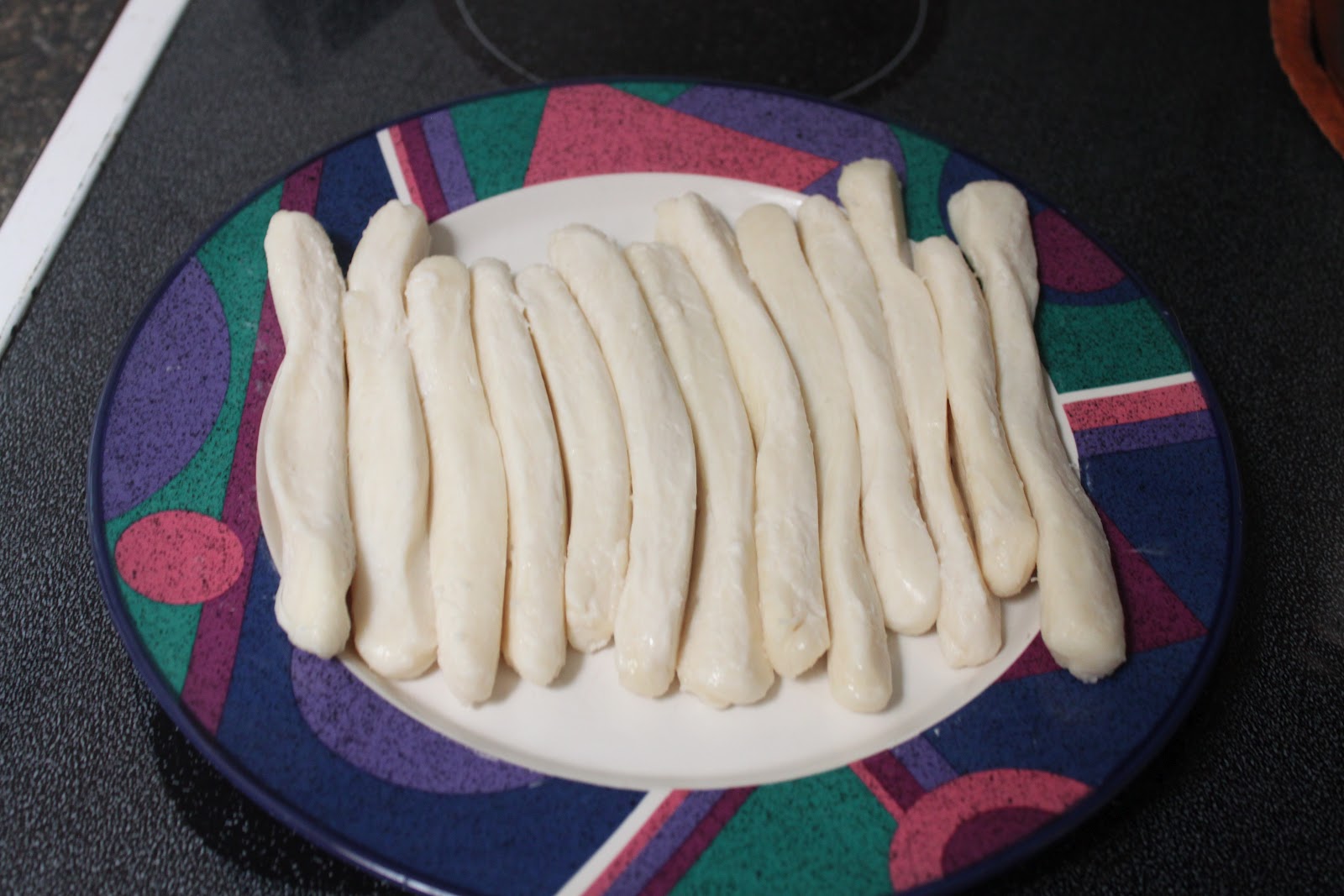This image features a single, colorful plate centered on a shiny black surface, likely a glass stove top with a gray, speckled pattern and partially visible black heating elements. The plate, artistically adorned with a vibrant array of pink circles, half-blue circles, aqua sections, purple stripes, teal, maroon, and dark green accents, creates a striking contrast against the white background at its center. Arranged neatly in a row on the white center of the plate are several long, white strips of what appears to be raw mozzarella cheese, resembling the size and shape of hot dogs or string cheese. The plate's position is close to the bottom of the image, slightly cut off, emphasizing its detailed design and the reflective surface beneath it, which suggests the setting is likely a kitchen.